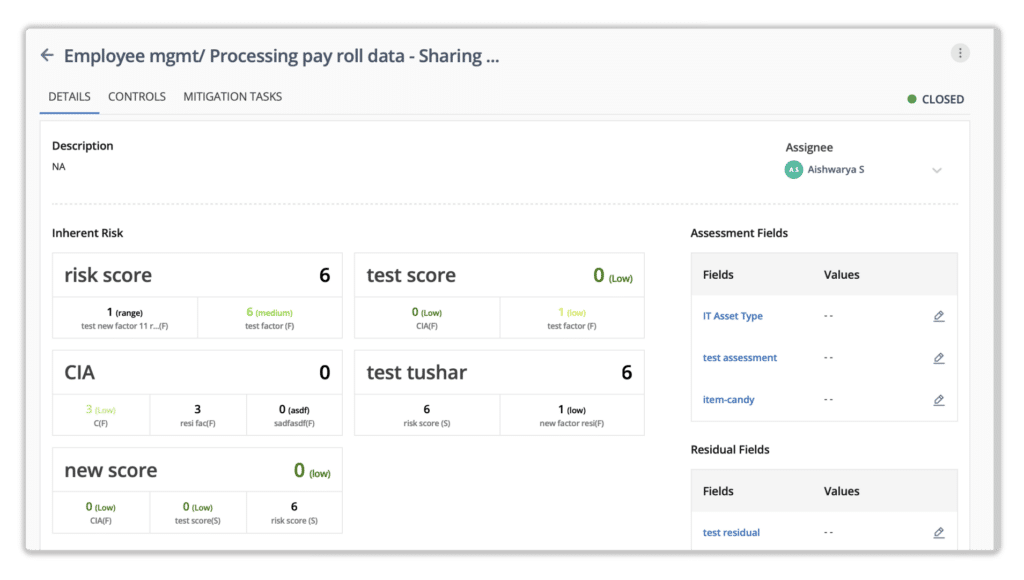The image features a light gray background with text and various sections organized in a structured format. At the top of the image, bold text reads "Employee Management/Processing Payroll – Sharing...". To the left of this title, an arrow points leftward. Below the title, several categorical labels are displayed horizontally: "Details," "Controls," "Mitigation," and "Tasks." 

On the right side of the image, a label marked "Closed" is prominent. Above this label, within a circle, there are three vertically aligned dots. Below this area, a small section provides a brief description labeled "N/A" and an "Assignee," followed by a person's name. The logo of the organization is nearby.

In the middle section of the image, the words "Inherent Risk" are displayed prominently. This section contains various metrics, including a "Risk Score," "Test Score," and "CIA Section" displayed in black text and numbers. Additionally, there is a mention of "SHAR" and a "New Score."

On the right, another section titled "Assessment Fields" is encased in a gray bar with black lettering. Beneath it, in blue text, difficult-to-read labels include "IT Asset Type," "Test Asset Access Management," and "Item Candy." This portion also lists "Residual Fields" with corresponding "Fields and Values" alongside "Test Residual."